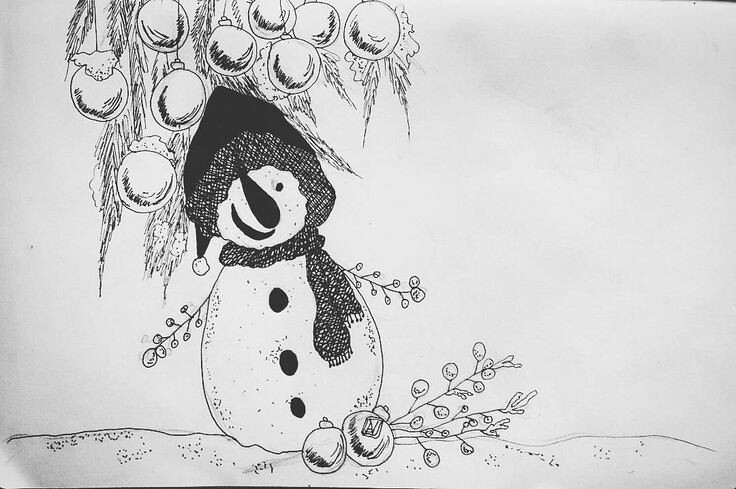This drawing on white paper features a charming snowman, meticulously rendered in pencil and then enhanced with pen. Faint eraser marks hint at the careful planning of the original sketch. The snowman is adorned with a cozy scarf and a festive hat, his face animated with a cheerful smile. Buttons march down his round body, adding to his traditional look. Surrounding him are a couple of Christmas ornaments scattered on the ground, along with some sprigs of holly berries. The upper part of the image is framed by boughs of a fir tree, from which various ornaments dangle, adding a festive touch. Despite being a monochromatic piece, the drawing captures the essence of holiday cheer. The quality of the artwork suggests it was created by someone with a decent level of skill, though not necessarily a professional artist.